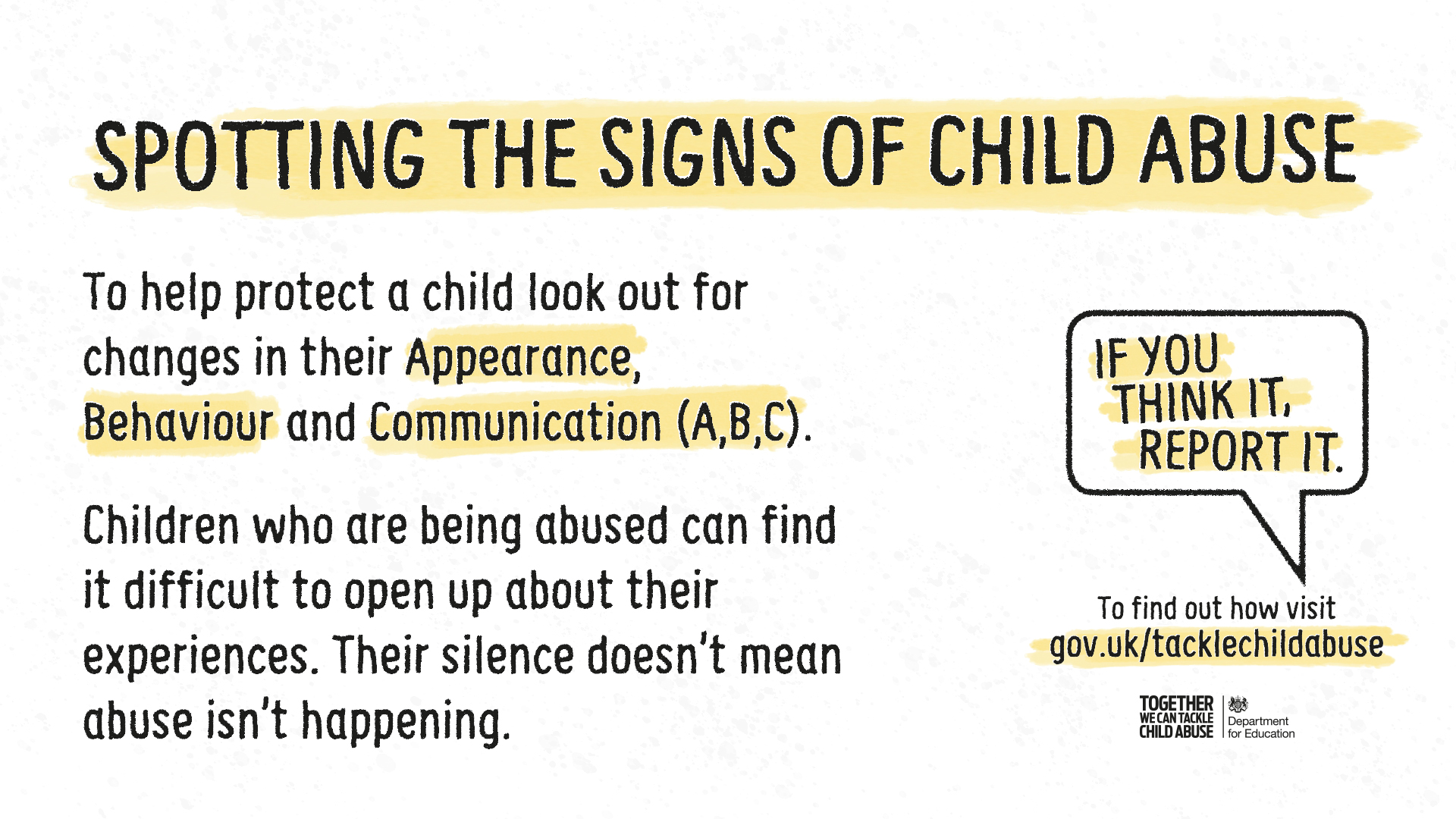The image is a public service announcement flyer from the UK, sponsored by the Department for Education. The background is tan with black lettering and organized sections. The top of the flyer prominently displays the heading "Spotting the Signs of Child Abuse." Below this, there are two important paragraphs, each on the left side. The first paragraph emphasizes: "To help protect a child, look out for changes in their appearance, behavior, and communication (ABC)." These words, "appearance, behavior, and communication," are highlighted in yellow. The second paragraph explains that "children who are being abused can find it difficult to open up about their experiences. Silence doesn't mean abuse isn't happening." To the right of the flyer, there is a speech bubble with the words, "If you think it, report it." Below the speech bubble is an arrow pointing to the directive: "To find out how, visit gov.uk/tacklechildabuse," highlighted in pale orange. At the bottom right corner of the flyer, it states, "Together We Can Tackle Child Abuse," accompanied by the Department for Education's logo.